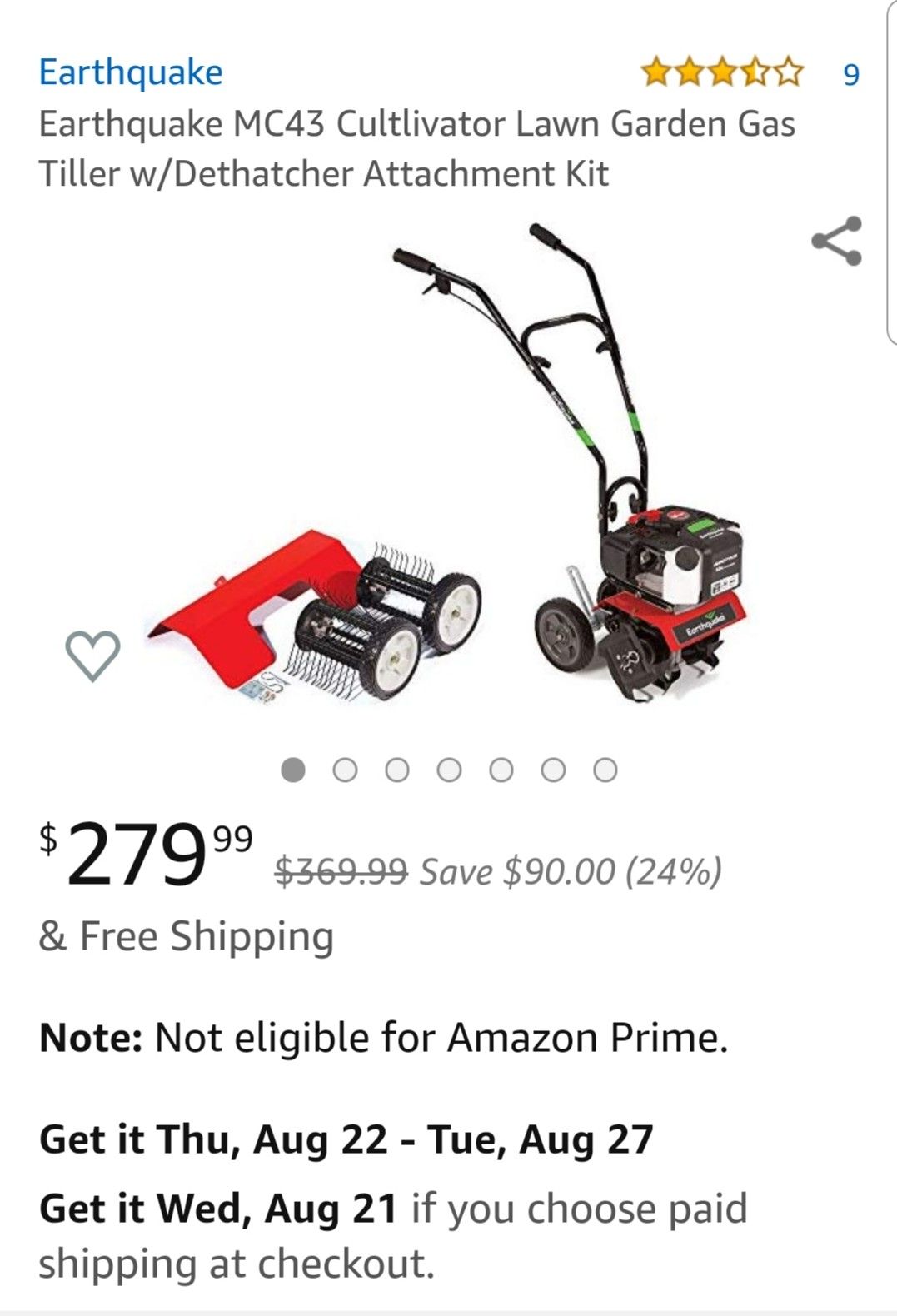The image is a screenshot with a white background featuring an advertisement for an "Earthquake MC43" cultivator. Described as a lawn and garden gas tiller with a width detacher attachment kit, the product is priced at $279.99, marked down from $369.99, offering a discount of $90 (24% off). The product image shows it has a rating of 3.5 stars. Additionally, the ad highlights free shipping, but notes that the item is not eligible for Amazon Prime. Delivery dates are specified as between Thursday, August 22 and Tuesday, August 27, with expedited shipping available for arrival by Wednesday, August 21 if paid at checkout. The image also features seven status circles, with the first one in gray and the remaining six in white.